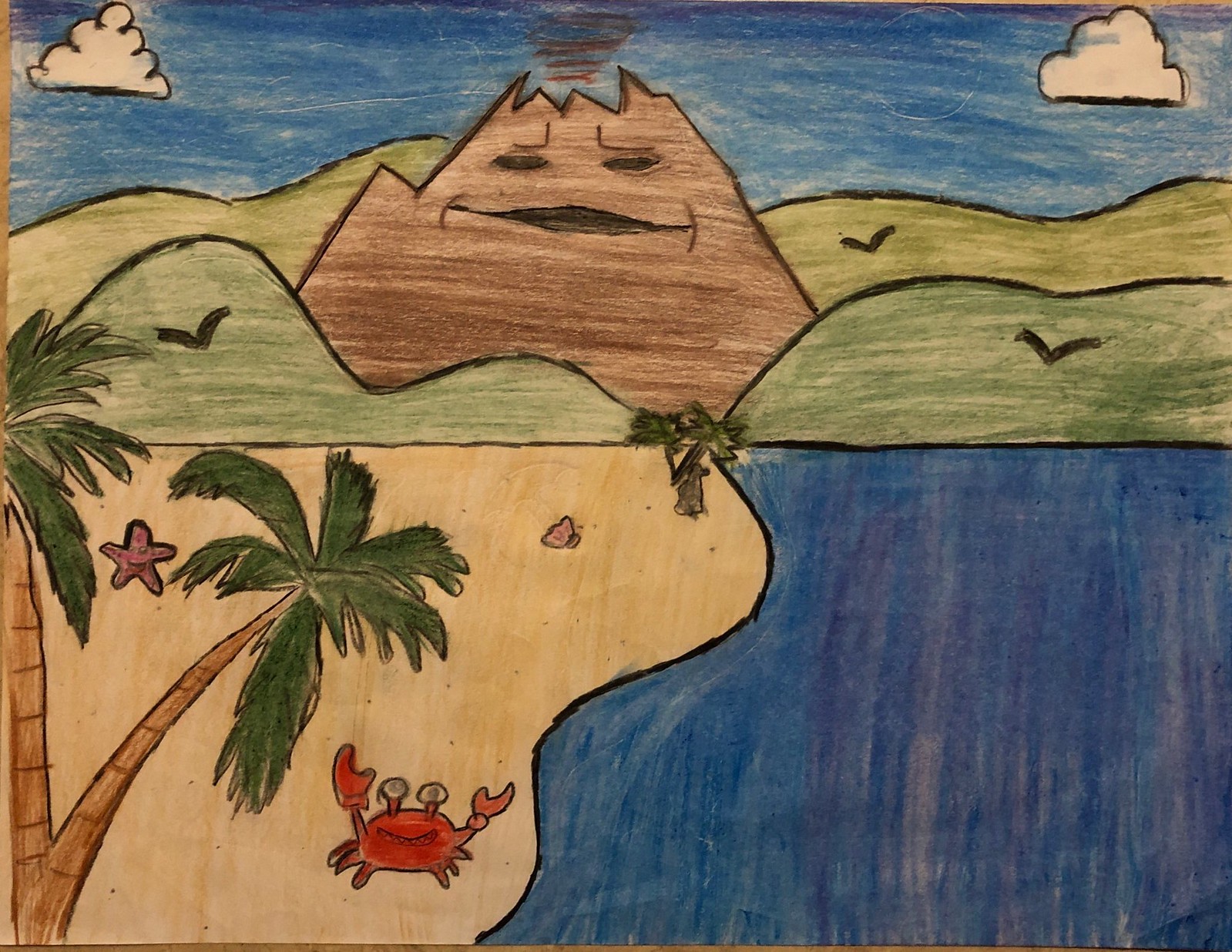In this intricate drawing, a vividly detailed tropical beach scene unfolds, dominated by a quirky, anthropomorphic volcano in the background. The lower right section features vibrant blue water with a gentle wave, seamlessly blending into the lower left, where a sandy beach stretches out. A graceful palm tree with a brown trunk and lush green leaves curves elegantly from the bottom left corner. Nestled beside it, a tiny, red crab scuttles close to both the tree and the water's edge.

Nearby, a delicate starfish lies between the tree trunk and the center of the beach, accompanied by a small clamshell further in the background. Another palm tree stands proudly near the center of the image, providing a sense of balance and symmetry.

Beyond these beachside details, a series of verdant green hills roll gently upwards, dotted with tiny birds soaring in the sky. The most striking feature is the volcano in the distance, which not only looms majestically over the landscape but also possesses a whimsical personality, complete with expressive eyes, eyebrows, and a cheerful mouth. This imaginative depiction blends nature and fantasy, creating a delightful and engaging scene.